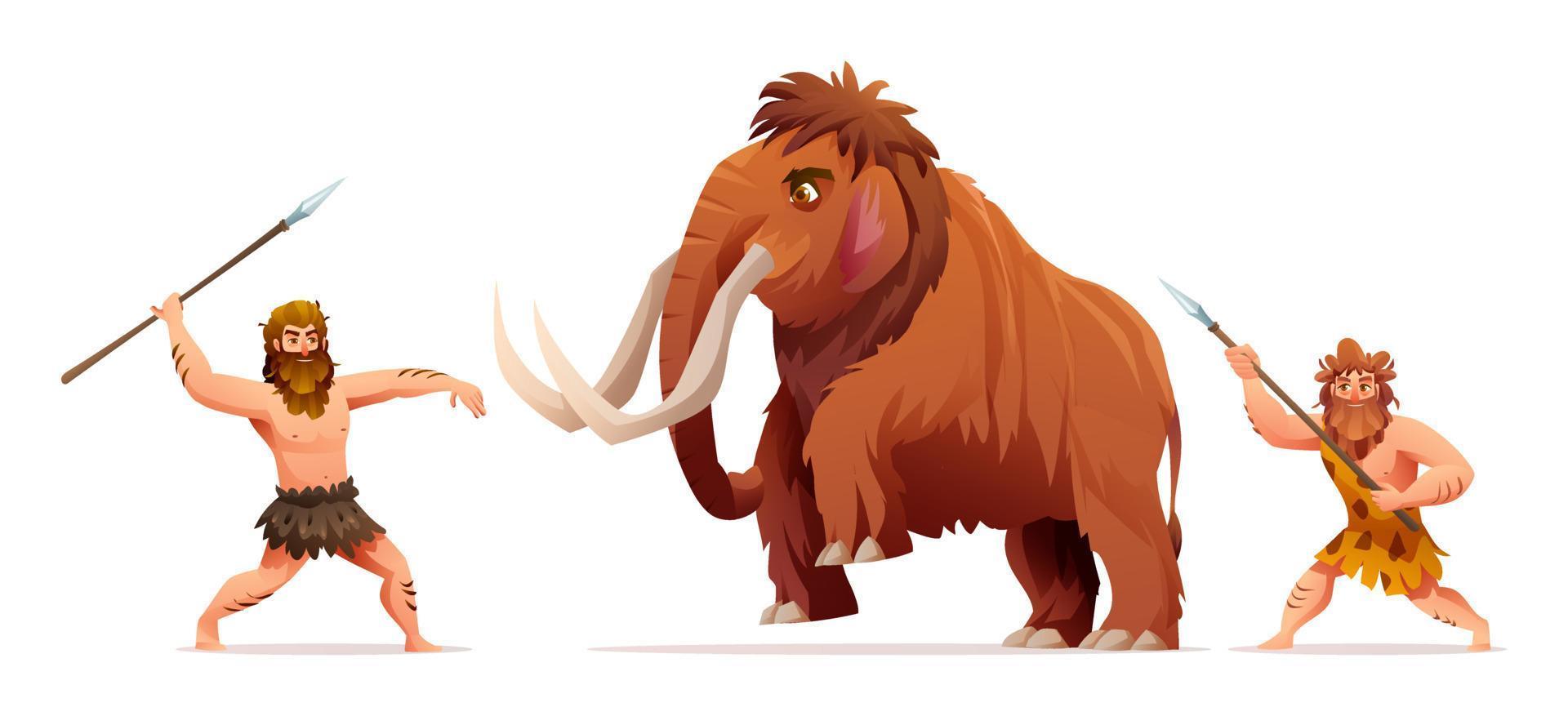This detailed cartoonish drawing depicts a dramatic scene where two muscular, young cavemen are attacking a large woolly mammoth with spears. The mammoth, standing at the center of the white background image, is a prominent light brown color with darker brown fur accentuating its neck and back. It boasts long, curving white tusks and a lengthy trunk hanging down. Its left front leg is raised, as if preparing to charge. 

On the left, a caveman with a bushy beard and abundant hair is poised to throw his spear. He wears a gray skirt and displays a belt with dark fur around his middle. To the right of the mammoth, the second caveman, equally bearded and muscular, wields his spear high, clad in a yellow and brown tunic that drapes over one shoulder. Both figures, illustrated with shadowing that provides a 3D effect, emphasize their intent and vigor in this prehistoric confrontation. The tan line beneath them suggests the ground, while their spears, possibly tipped with materials like quartz crystal, hint at a resourceful adaptation.